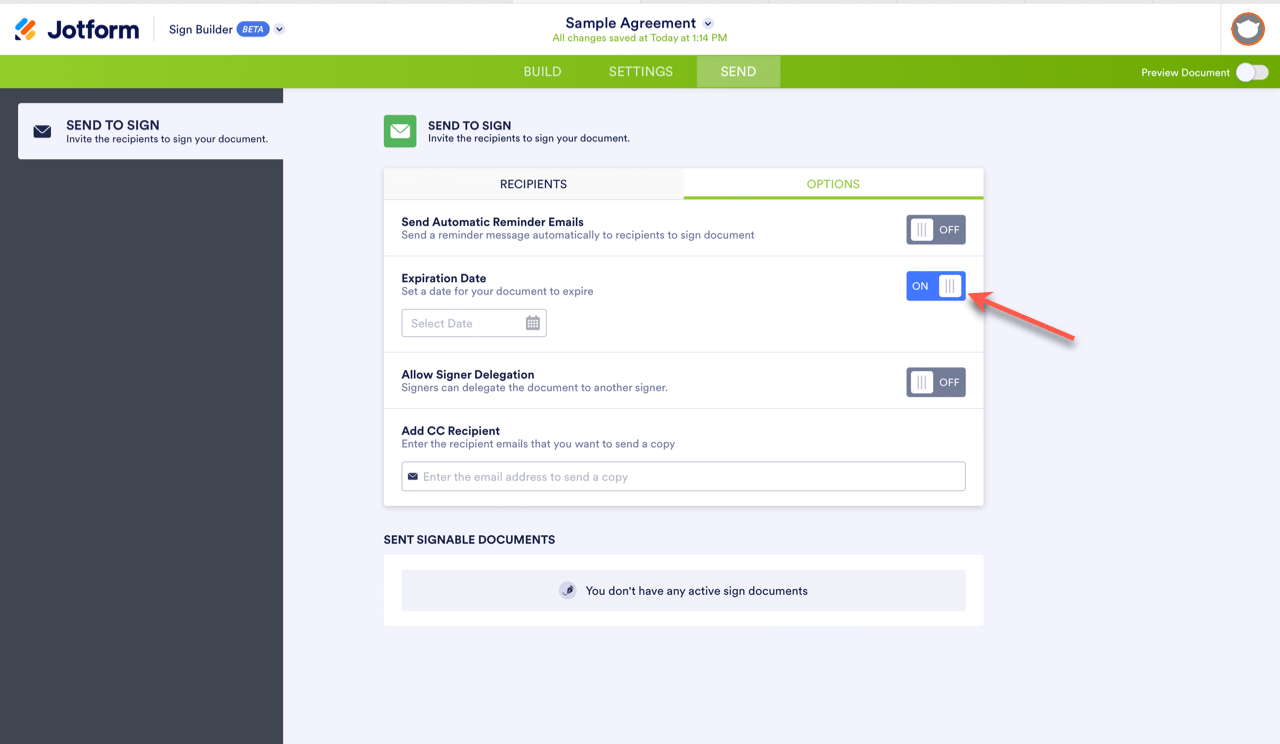This image is a screenshot of an online document signing platform, specifically showcasing JotForm's SignBuilder tool. The interface displays a draft titled "Sample Agreement," indicating it is set up for electronic signing. At the top left corner, the JotForm logo is prominently displayed, followed by the label "SignBuilder beta," highlighting that the tool is in its beta phase.

The title "Sample Agreement" is centrally positioned with a small icon confirming that all changes were saved at 1:14 PM on the same day. On the top right, there is a toggle for previewing the document, which appears to be switched on, indicating that the current view is the preview mode.

The top center of the interface features three main tabs: "Build," "Settings," and "Send." The "Send" tab is currently active and highlighted in green, suggesting that the user is in the process of configuring the document for sending. The layout and details provide a comprehensive overview of the document signing setup within the JotForm's SignBuilder tool.